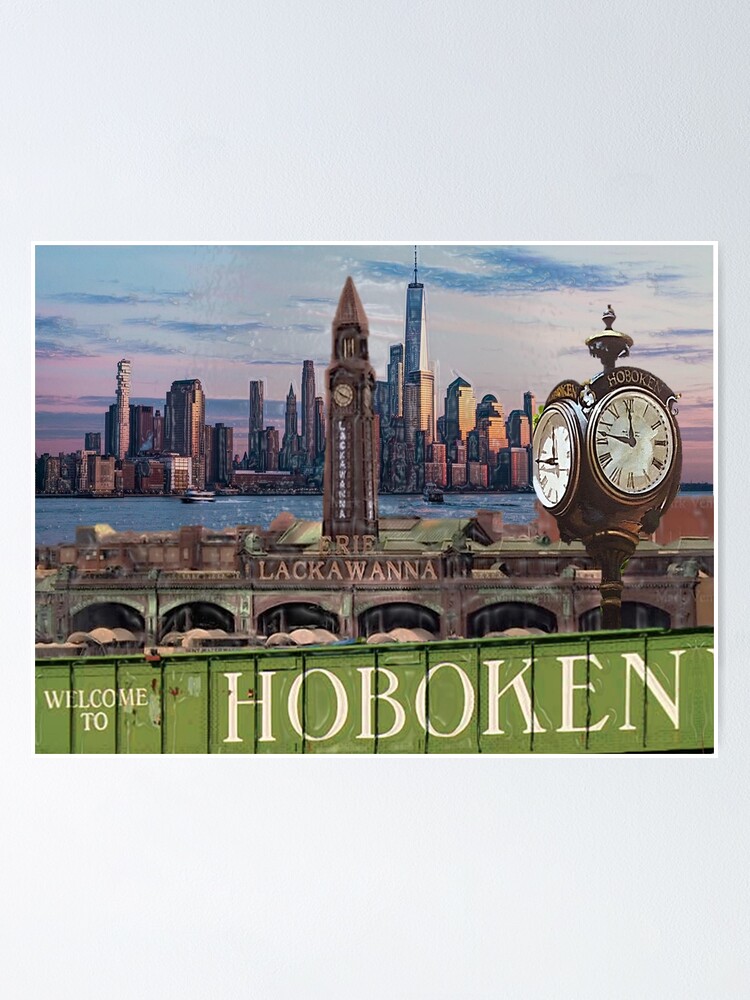The image is a detailed and colorful painting, likely done in acrylic or watercolor, portraying a vibrant scene of Hoboken, New Jersey. Dominating the foreground is a green banner with large white text that reads "Welcome to Hoboken," which could either be part of a train car or the side of a railroad bridge. Above this, an old-fashioned street clock with multiple faces rises prominently, reminiscent of a lamppost. Directly behind the clock tower, there is a historic, long, low building adorned with broad arches and marked with the words "Lackawanna" and "Erie Lackawanna," suggesting it might be a train depot. Towering above this structure is the clock tower, also labeled "Lackawanna," featuring a peaked, spire-like top with an analog clock visible on its side. Further in the background, a calm body of water stretches across the scene, leading to a distant cityscape. The skyline, likely of Manhattan, is depicted with tall skyscrapers set against a serene pastel-colored sky, casting an atmospheric glow over the entire composition. The overall vertical layout of the image, along with its rich details and lively colors, brings the essence of Hoboken to life, making it appear as a welcoming postcard capturing the essence of the city.